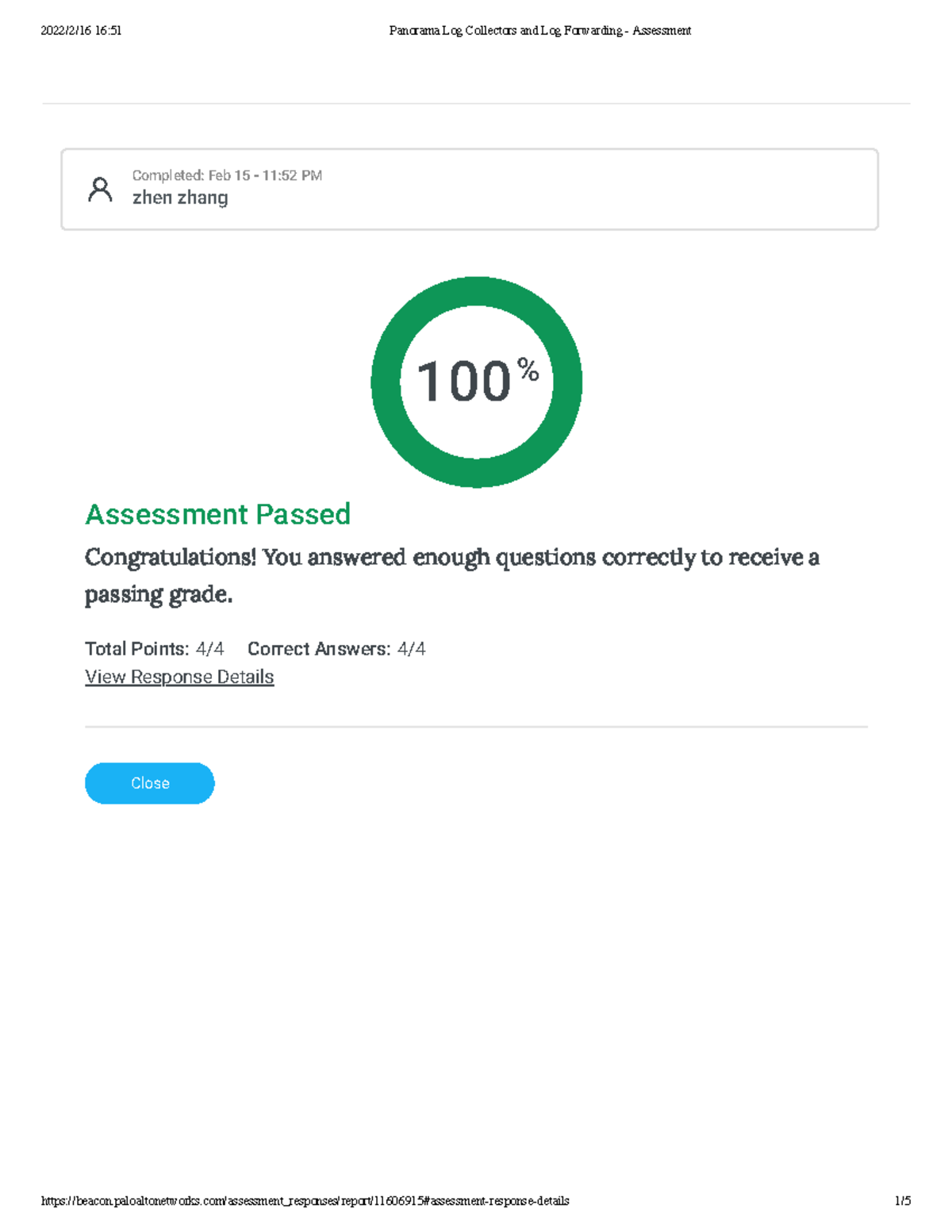This detailed caption corresponds to the provided image: 

The screenshot shows a final grade page from an assessment website or application. The interface features a clean, predominantly white design with minimal black text and green highlights. Positioned at the top of the page, the black text indicates that the assessment has been completed, alongside the date and the participant’s name. Dominating the center is a prominent green-banded circle with a white interior, displaying a bold "100%" in black. Beneath this, green text states "Assessment Passed," followed by black text congratulating the individual with the message: "Congratulations, you answered enough questions correctly to receive a passing grade." Further details are provided with "Total Points: 4 of 4" and "Correct Answers: 4 of 4," reinforcing the achievement. There is an option to view response details via a link. At the bottom of the page, a blue, rounded rectangular button labeled "Close" allows the user to exit the screen. The page is designed with ample blank space, accompanied by a header, footer, date, and an unreadable URL at the very bottom, contributing to its uncluttered and user-friendly appearance.